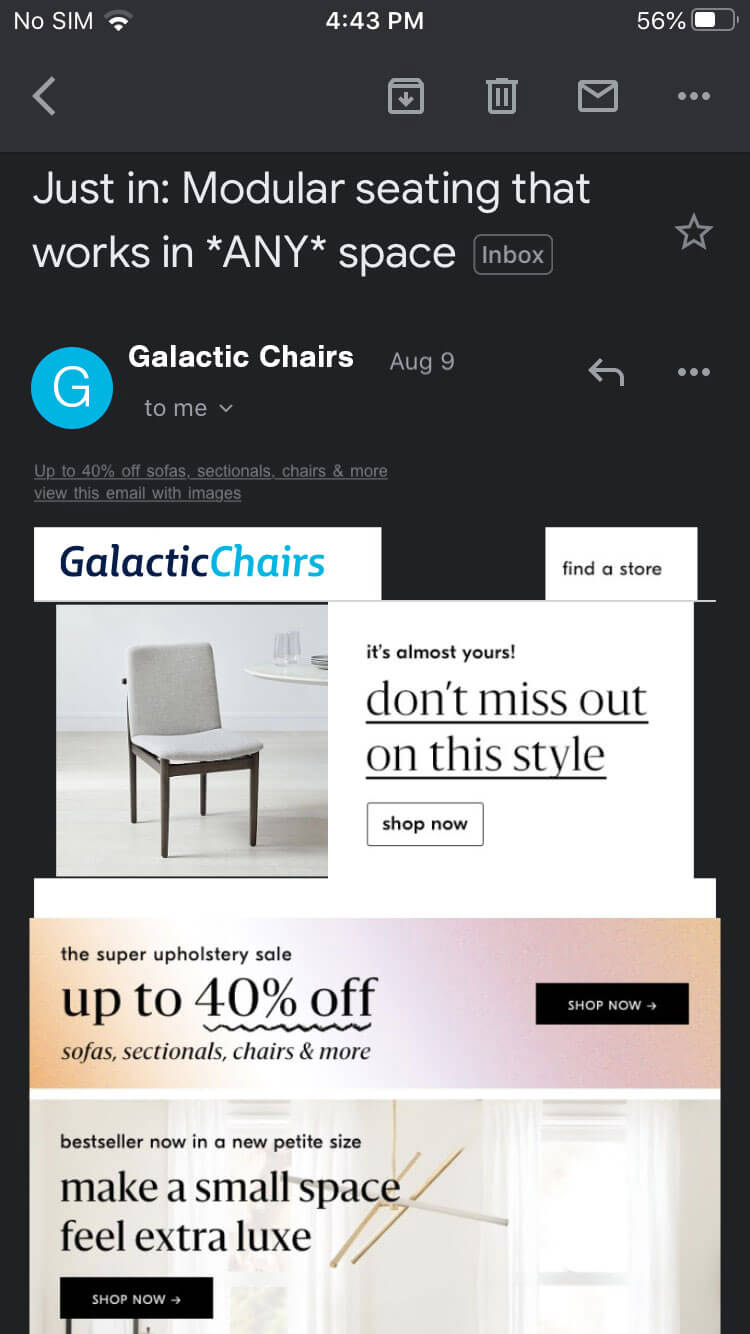In this image, we see a screenshot dominated by a primarily black background. At the top, we notice a dark gray header with white text. In the upper left corner, there is an indication that there is no SIM card inserted, and the Wi-Fi is on. In the center, the time displays 4:43 PM. To the right, there's a battery icon showing 56% charge. Below this header, set against a black background, is an icon of a trash can, symbolizing the delete option, next to an envelope icon indicating messages.

Further down, a bold text reads: "Modular seating that works in any space." To the right, there's an "Inbox" button. Underneath, another headline reads: "Galactic Chairs," accompanied by a blue circle with the letter "G" inside. Another offer below states: "Up to 40% off sofas, sectionals, chairs, and more." A link following this text invites viewers to "View this email with images."

Beneath the text, there's a color photograph of a sleek white chair with wooden legs, lacking armrests. To the right of the chair, the text advises: "It's almost yours, don't miss out on this style." At the very bottom of the screenshot, there's a white "Shop Now" button encouraging immediate action.